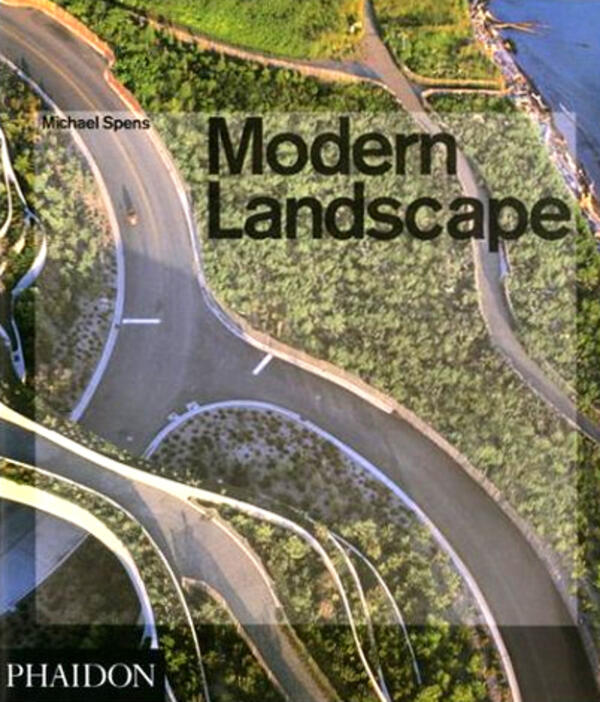This detailed aerial photograph serves as the cover of a book titled "Modern Landscape" by Michael Spence, published by Phaidon. The photo, taken on a clear day, showcases a complex overhead view of a landscape featuring prominent roadway elements. 

Central to the image is a large, gray concrete or asphalt highway shaped like an upside-down "Y," adorned with white borders and a central stripe. This highway runs diagonally from the top left to the bottom right of the image. To the right of this primary road is a lush, green expanse of trees, beyond which lies a narrower, winding one-lane road and a stretch of grass leading to the ocean visible in the upper right corner.

The photograph is digitally enhanced to accentuate its vibrant colors and intricate details. Superimposed on the photo within a semi-transparent white square are the title and author's name, written in small, black Arial-like font: "Michael Spence" at the top left and "Modern Landscape" on the right side. At the very bottom left corner of the image is a black rectangle with white lettering spelling out "P-H-A-I-D-O-N." The cover encapsulates the intersection of natural and man-made landscapes, emphasizing the harmonious yet complex relationship between highways and their verdant surroundings.